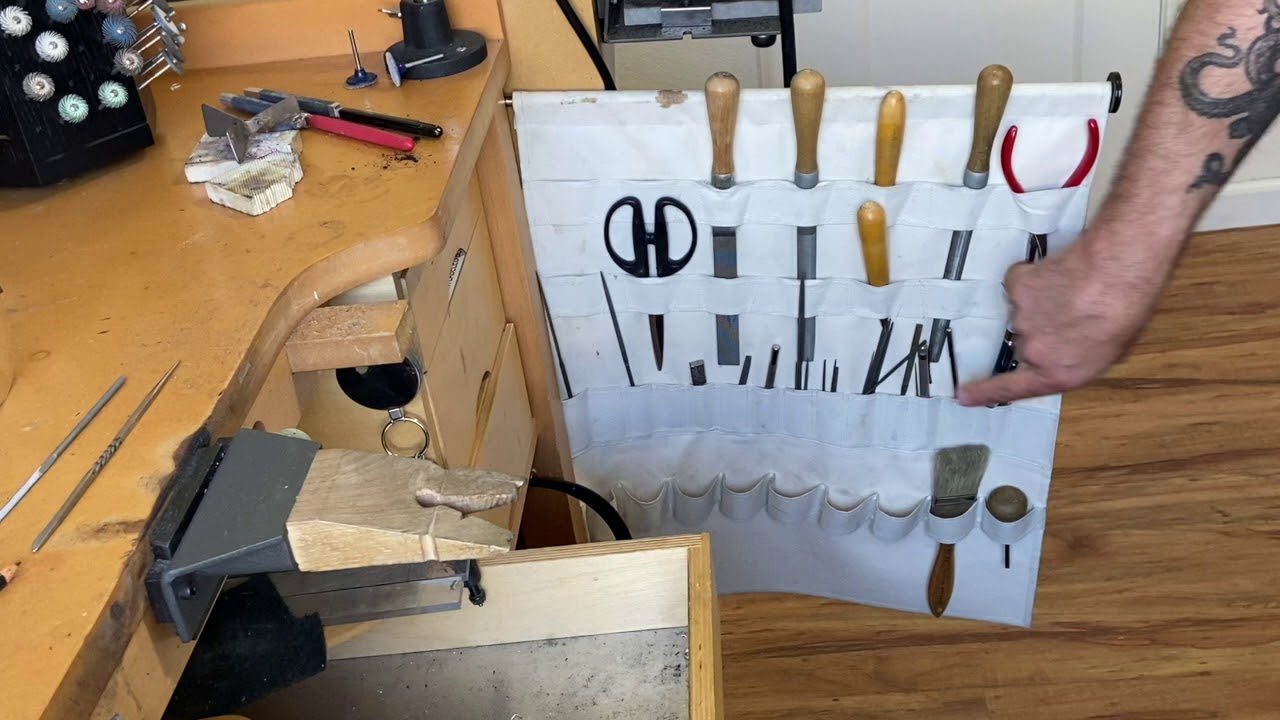This detailed photograph showcases a bustling workshop, likely a jeweler's workbench, emphasizing a meticulously arranged workspace. On the left side, a brown wooden workbench is clearly visible, complete with various tools such as grinders, drills, Dremel tools, and files. A jeweler's vise and some closed drawers add to the organized chaos of the bench area. Prominently, a white canvas tool organizer hangs horizontally, extending out from the workbench. This organizer boasts about seven sleeves per row over four rows, neatly housing an array of tools including scissors, chisels, sanding tools, pliers, paintbrushes, and files. On the right side of the image, a man's tattooed arm—possibly depicting an octopus—extends into the frame, pointing at a particular tool in the organizer. The arm and the action of pointing at a specific tool draw attention to the detailed and carefully curated workspace, reflecting the precision and craftsmanship inherent in the jeweler's trade.